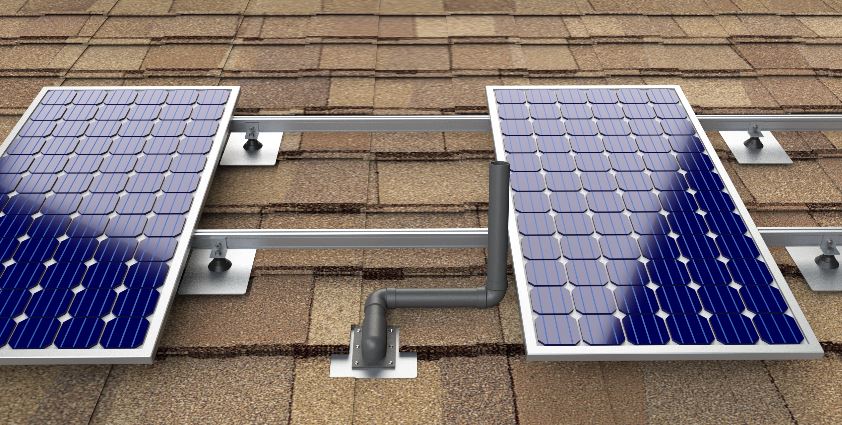This is a horizontally aligned, wide close-up image of a rooftop taken during the daytime. The roof is covered with alternating medium brown and dark brown shingles. Prominently featured on the roof are two vertical rectangular solar panels, one on the left and one on the right, held in place by horizontal metal bars. Between the solar panels, a dark gray L-shaped pipe runs vertically. On the right side of each solar panel, there are small square metallic boxes with knobs protruding from them. The solar panels themselves have light gray borders and are composed of numerous tiny squares with vertical blue lines. The daytime light reflects off the blue and silver elements of the panels and surrounding fixtures, highlighting their details against the earthy tones of the shingles.